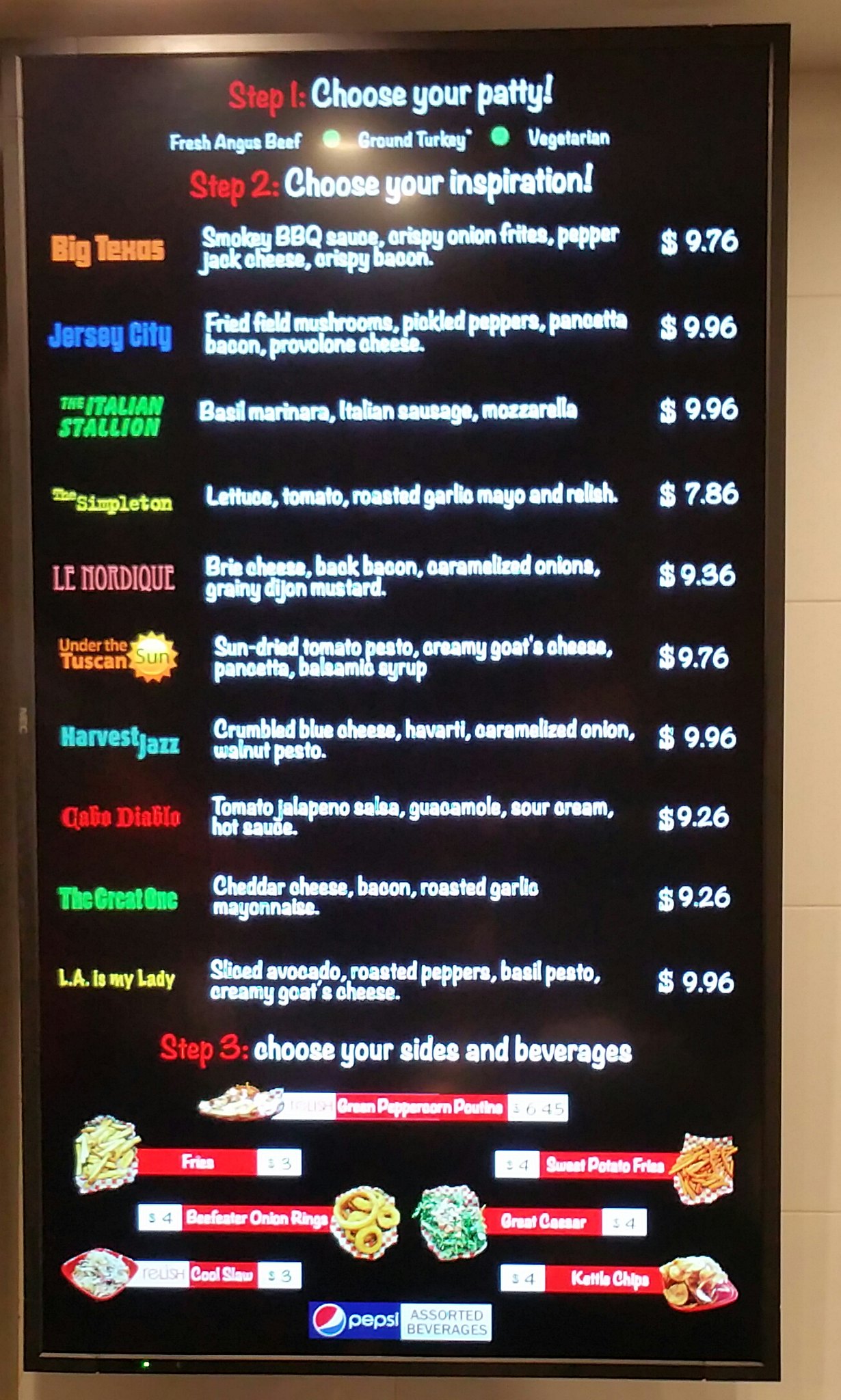A vibrant, brightly-lit poster on the wall captures attention with its colorful LED-enhanced display, guiding diners through a customizable burger experience. The process is clearly outlined in three steps, beginning with "Step 1: Choose Your Patty," offering options such as fresh Angus beef, ground turkey, or a vegetarian substitute. Moving on to "Step 2: Choose Your Inspiration," customers can select from themed combinations, like "Big Texas," featuring smoky barbecue sauce and crispy onion fries, or "LA is My Lady," with sliced avocado, roasted peppers, and basil pesto. Finally, "Step 3: Choose Your Sides and Beverages" provides a range of choices, including fries, sweet potato fries, and Caesar salad. The total cost for most meals hovers around $9.76, suggesting this menu might be a bit dated but still offers a detailed and enticing guide through the dining options available, reminiscent of the Five Guys burger experience.